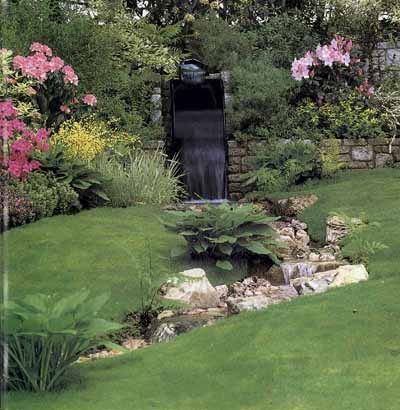This is a square photograph depicting a serene garden scene centered around a water fixture. In the foreground, a grassy area dominates the bottom right corner, while a broad-leaved green plant flourishes in the bottom left. A gully, resembling a natural creek with rocks, threads its way from the bottom left upward, curving to the right before bending back to the left as it ascends. Water can be seen flowing over the rocks, suggesting a gentle stream. 

Midway up the image, there are more grassy patches on both sides of the creek. On the left bank, a green shrub clings to the edge, and on the right bank, additional grass stretches toward the center. Dominating the background is a waterfall cascading from a black, rectangular fixture topped by an enigmatic sphere. This waterfall flows into the creek below, creating an idyllic water feature.

To the left of the fixture, flowering bushes with pink and yellow blossoms thrive, adding a burst of color. On the upper left side, a mix of bushes and trees further enriches the scene, with pink, purple, and yellow flowers interspersed among the greenery. On the right side, another array of bushes is flecked with white and pink flowers, backed by a stone wall that runs from right to left behind the waterfall. This stone wall continues off the image, adding a structured element to the natural landscape, while the incline behind it supports more blossoming bushes and trees, enveloping the garden in lush, layered beauty.